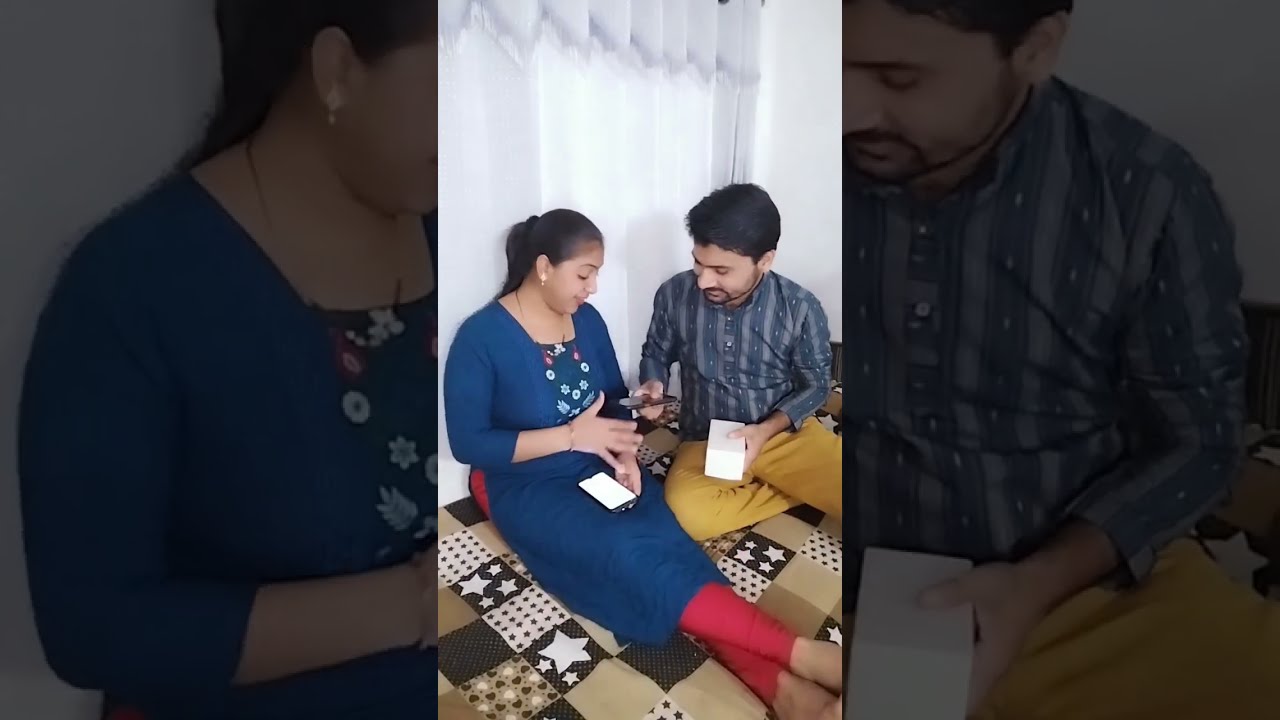The image is a wide rectangular frame featuring a central tall rectangular photograph of a couple and this central image is flanked on both sides by dark, zoomed-in close-ups of the same photograph. The couple is seated on a patchwork quilt that covers a bed. The quilt is composed of various shades of brown, white, and tan, featuring designs like stars, polka dots, and hearts.

On the left side of the photograph is a woman with black hair tied back in a ponytail, dressed in a blue dress with a floral wreath pattern and red leggings, stretching her legs outward. She holds a cell phone on her lap with her fingers poised just below it, while her gaze is directed at another cell phone held by the man sitting next to her.

The man, positioned to her right, has short black hair and wears yellow pants and a blue striped shirt. He is holding his cell phone out, showing something on the screen to the woman. The detailed close-ups of the photograph emphasize the couple's interaction and the intricate patterns on the quilt beneath them.